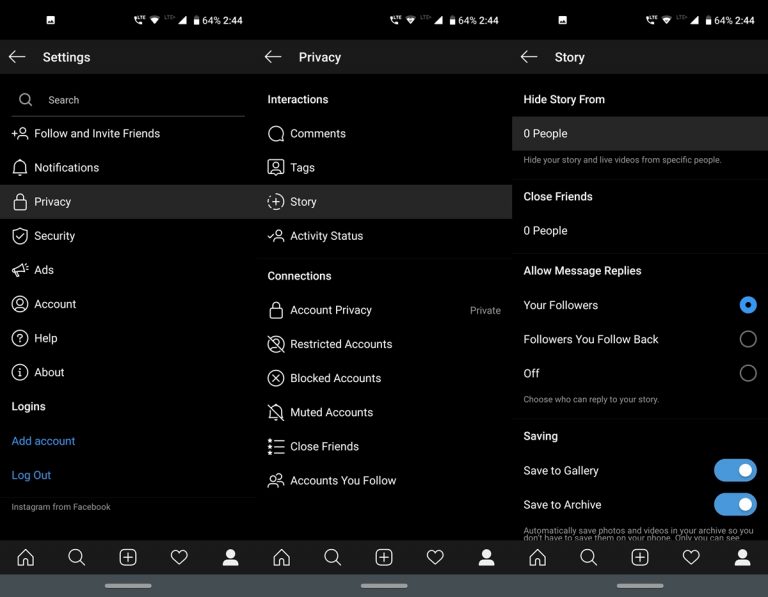The image is a square with a black background, displaying a detailed chart that resembles a tablet screen turned on its side, divided into three columns. 

**First Column:** 
- At the top right of the first column, it shows a battery icon indicating 64% and a timestamp of 2:44 PM.
- Beneath this, there's a gray stripe labeled "Settings" followed by a search bar and a list of options, including:
  - Follow
  - Notifications
  - Privacy
  - Security
  - Ads
  - Account
  - Help
  - About
  - Logins
- Highlighted in blue are "Add Account" and "Logout," suggesting these are clickable links.
- The "Privacy" option is selected, indicated by its light gray background.

**Second Column:**
- Similar to the first, it shows a timestamp of 2:44 PM.
- A dark gray stripe labeled "Privacy" is at the top, beneath which are options:
  - Interactions (Comments, Tags, Story Activity, Status)
  - Connections (Account Privacy, Restricted Accounts, Blocked Accounts, Muted Accounts, Close Friends, Accounts You Follow)
- The "Story Activity" option is highlighted with a gray background.

**Third Column:**
- The top of this column also shows a timestamp of 2:44 PM.
- A light black stripe labeled "Story" is at the top, followed by:
  - "Hide Story From" with zero people selected
  - "Hide Your Story and Live Videos from Specific People" with no blocks
  - "Close Friends" set to zero
  - "Allow Message Replies," with toggles showing:
    - Your Followers (blue)
    - Followers You Follow Back (white/translucent off)
- The saving options were toggled on:
  - Save to Gallery
  - Save to Archive